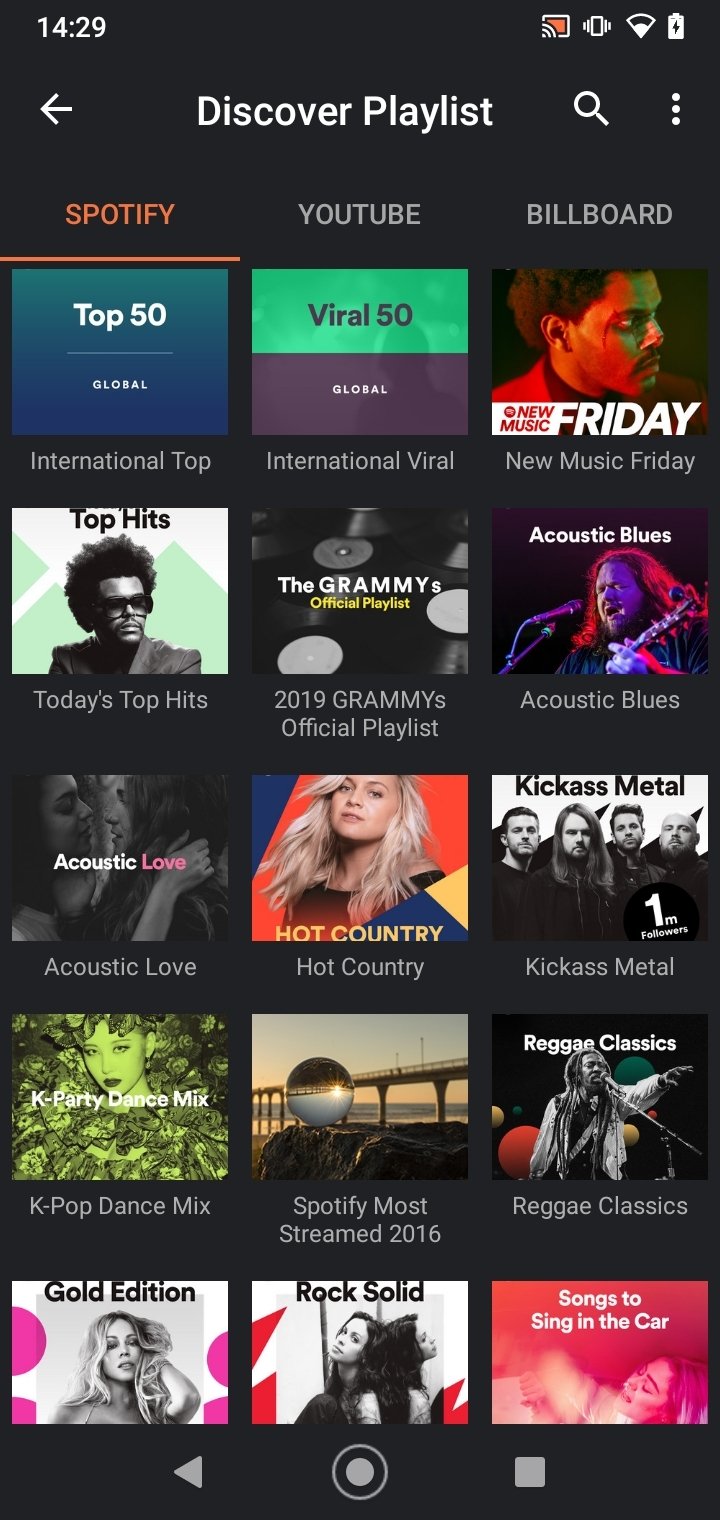A screenshot captured on a smartphone displays a music website interface with a sleek black background and white text. At the top-left corner, the time reads 14:29, and the status bar includes icons for cell signal, battery life, and connection status. Below the time, the header features "Discovery Playlist" in bold white letters, flanked by a back-arrow icon, a search icon, and a three-dot menu icon.

The main content is organized into three vertical columns labeled Spotify, YouTube, and Billboard. Each column showcases five playlists with their respective titles and thumbnail images.

In the Spotify column, the playlists listed are:

1. International Top 50 Global
2. Today's Top Hits
3. Acoustic Love (accompanied by a relevant picture)
4. K-Pop Dance Mix (featuring an image of a woman in green)
5. Gold Edition (partially visible with a woman's image at the top)

In the YouTube column, the playlists are:

1. Viral 50 Global
2. The Grammy’s Official Playlist
3. Hot Country
4. Spotify Most Streamed 2016
5. Rock Solid

In the Billboard column, the playlists featured are:

1. New Music Friday
2. Acoustic Blues
3. Kick-Ass Metal
4. Reggae Classics
5. Songs to Sing in the Car

Each playlist is represented by a box containing various images corresponding to the playlist’s theme. The clean layout and contrasting colors make it easy to navigate through the diverse music choices.